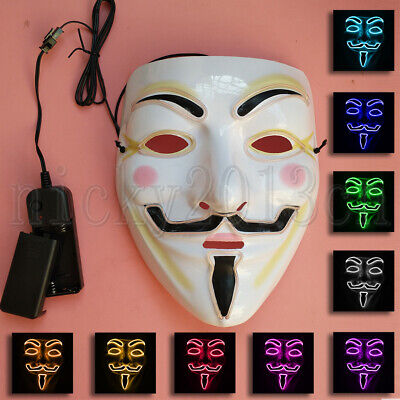This detailed photograph features a haunting, white Guy Fawkes mask with several striking and exaggerated facial features. The mask has red eye cutouts, a black handlebar mustache, sharp black goatee, and thick black eyebrows. Its cheeks are adorned with circular pink dots, adding to its eerie appearance. A black electronic cord is attached to the left side of the mask, connected to a battery port, which likely powers the LED lights within the mask. Surrounding the mask is a grid of black square panels depicting the mask's facial features—eyebrows, eyes, beard, and mustache—illuminated in a spectrum of colors. These squares frame the pink surface on which the mask rests, with five squares along the bottom displaying the mask in orange, yellow, red, pink, and purple hues. To the right are four more squares showcasing the mask in light blue, dark blue, light green, and white. Each colored panel casts the mask in a different light, enhancing the overall spooky and electrifying effect.